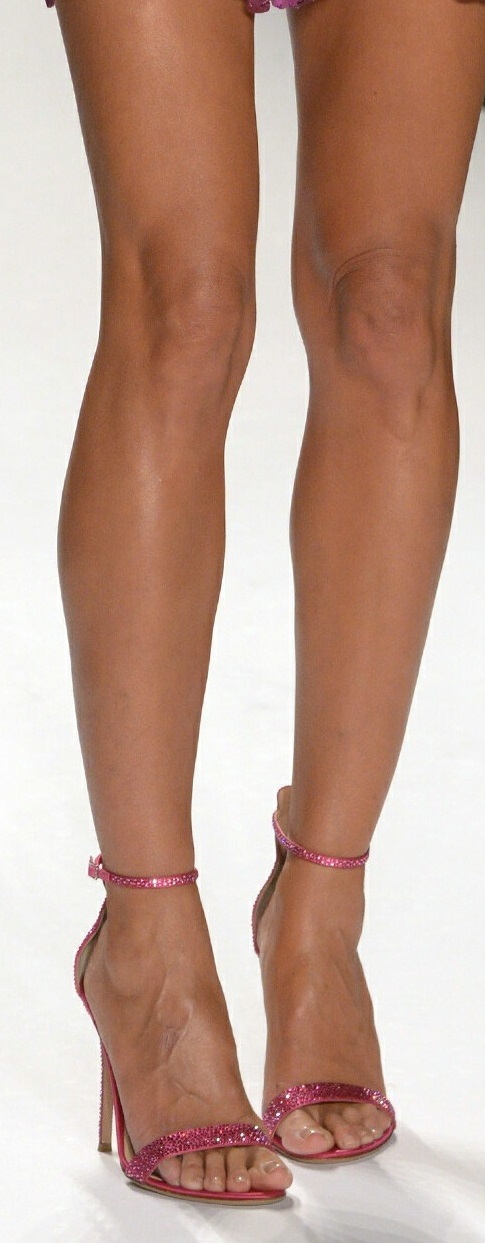This close-up color photograph showcases a woman’s legs from mid-thigh down to her feet, highlighted against a stark white background. Her bare legs appear smooth, likely recently shaved or waxed, with noticeable, slightly asymmetrical knees—one smoother, the other knobbier with faint wrinkles above it. At the top, the edge of a pink garment, possibly a dress or shorts, becomes visible. Her feet are adorned with pink, sparkly high-heeled shoes, featuring two straps: one around the ankle and one over the toes, giving the impression of being encrusted with rhinestones or sequins. The shoes' sheen is accentuated by her clear, reflective toenail polish. The shoes' and feet's shadows suggest the light source is positioned behind her.